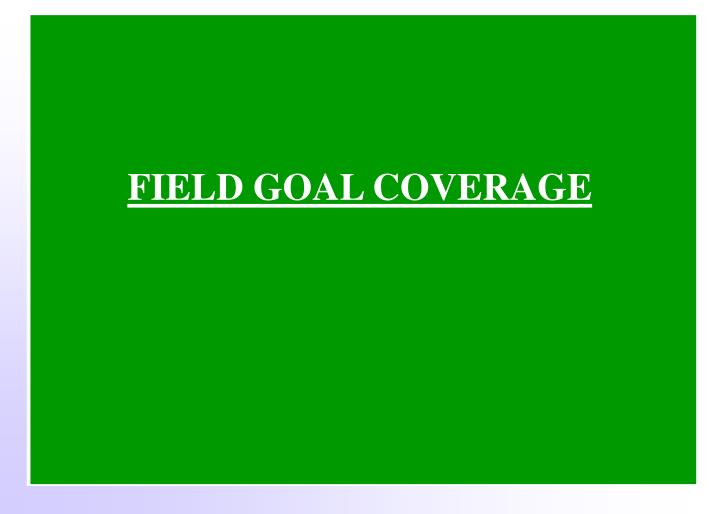This image is a simple graphic, resembling something that might be used in a PowerPoint presentation. It features a solid lime green background with a gradiated blue border, noticeable primarily at the bottom left. In the center of the green background, slightly towards the top, there is white text in all capital letters that reads "FIELD GOAL COVERAGE." The text is underlined and is written in a serif font, possibly Times New Roman. There are no other objects or elements in the image, making it very straightforward and easy to read. The colors present are green, white, and blue, creating a clean and focused visual with a professional feel.